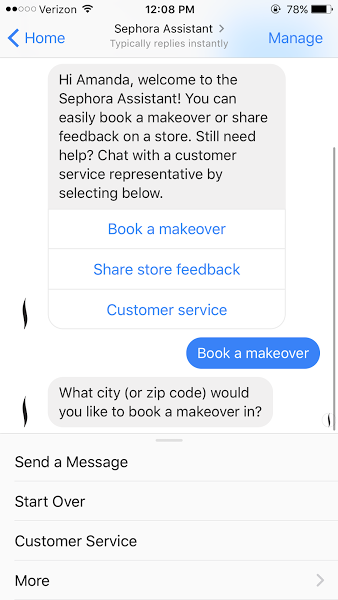This screenshot, taken on a mobile phone, showcases someone engaged with the Sephora Assistant chat interface. The top-left corner displays the phone’s signal strength with two out of five bars, alongside the Verizon carrier name and a Wi-Fi icon. Centrally positioned, the clock reads 12:08 p.m. On the top-right, there is a padlock icon and the battery status indicating 78% charge.

The interface features a blue back button and home button on the left, with a "Manage" option also displayed in blue on the right. The main content of the screen is a chat interaction with the Sephora Assistant, which prominently states, "Sephora Assistant typically replies instantly." Below, it greets the user with, "Hi, Amanda. Welcome to the Sephora Assistant."

The chat interface offers Amanda options to book a makeover, give store feedback, or connect with a customer service representative. She has typed "book a makeover," prompting the assistant to ask, "What city or zip code would you like to book a makeover in?"

Further interactive options are present at the bottom, including "Send a message," "Start over," "Customer service," and "More." The screen has a clean white background with the recognizable slender, wavy Sephora 'S' logo visible on the left side of some text elements. The bottom part of the screen is cut off, showing no navigation bar or additional content.